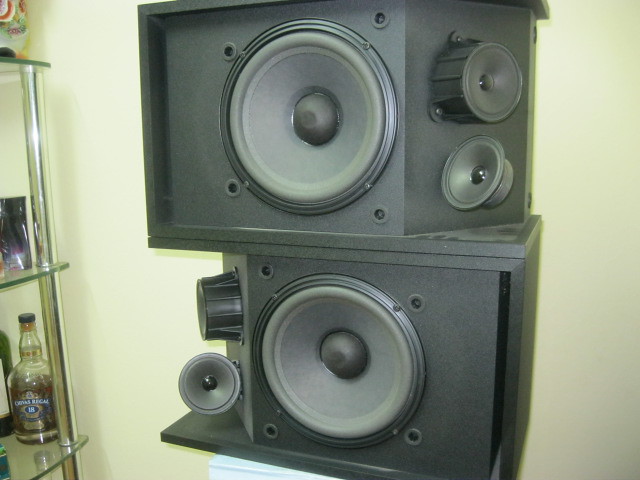The image captures a detailed scene featuring two professional, rectangular box speakers stacked on their sides in the middle of the frame. The bottom speaker is positioned with its topside facing left while the top speaker's topside faces right, creating a dynamic visual contrast. Each speaker showcases a central large woofer, a smaller tweeter at the top, and what appears to be a horn, providing a classic audio setup. Notably, there are several small circular elements near the speakers, possibly knobs or additional mini-speakers, adding to their intricate design. The speakers are housed in a somewhat dusty cabinet, suggesting age or infrequent use.

To the left of the speakers is a stylish glass shelf supported by a metal pole. The shelf holds an assortment of items, including liquor bottles and collectible glassware. One specifically identified item is an empty Chivas Regal whiskey bottle. An intriguing decorative piece that resembles a skull or face adds a unique touch, indicating this scene might be located in a used goods store or thrift shop. The background contrasts with a white wall, providing a neutral backdrop to the eclectic assortment on the shelf and the prominently featured box speakers.